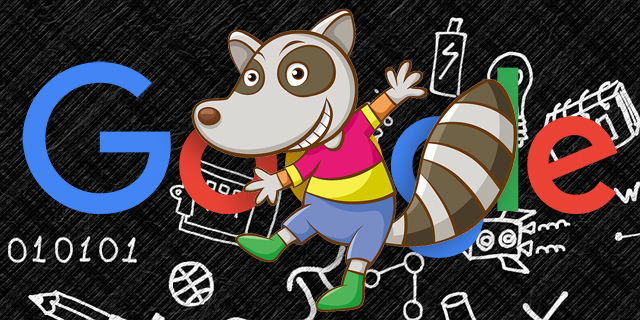The image is a computer-generated artwork depicting a cheerful raccoon standing in front of the word "Google," which is rendered in its iconic bright, primary colors on a black, subtly textured background. The raccoon, which has a grey and brown-striped tail, is anthropomorphized, wearing a vibrant pink and yellow striped shirt, blue shorts, and green shoes, with its arms outstretched in a welcoming pose. 

The word "Google" is partially obscured by the raccoon but can still be identified: the G is blue, the first O is red, the second O is yellow, the second G is blue, the L is green, and the E is a reddish-orange. Surrounding the Google logo are various childlike doodles in white, including a pencil, a basketball, the binary code "010101," a spiral notebook, a battery, a spaceship, and the π symbol, suggesting educational or playful themes. This detailed assemblage suggests that the image might be a decorative banner or poster, likely for one of Google's thematic promotions, perhaps related to learning or a special event.